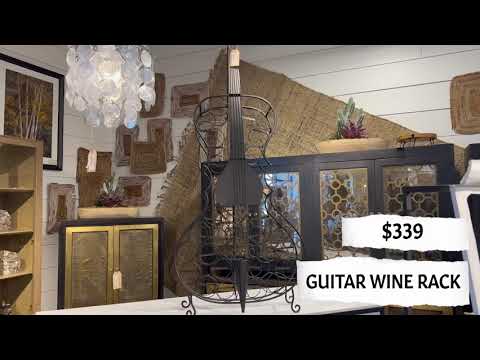The image presents a meticulously designed guitar-shaped wine rack, prominently displayed on a white table in what appears to be an antique or home decor store. The guitar wine rack, priced at $339 as indicated by the text in the lower right corner, features a black metal frame with circular openings for holding wine bottles and a detailed centerpiece resembling guitar strings. Surrounding this focal point are various antique furnishings: a black cabinet with mirrored and golden doors, an assortment of sculptures on bookshelves, framed artwork, decorative wooden blocks, and a modern chandelier hanging from the ceiling. The store's background is composed of white wooden plank walls adorned with various decorations, enhancing the vintage ambiance. The image is framed with black borders on the top and bottom, further emphasizing its purpose as a product image likely intended for social media marketing by a retailer.